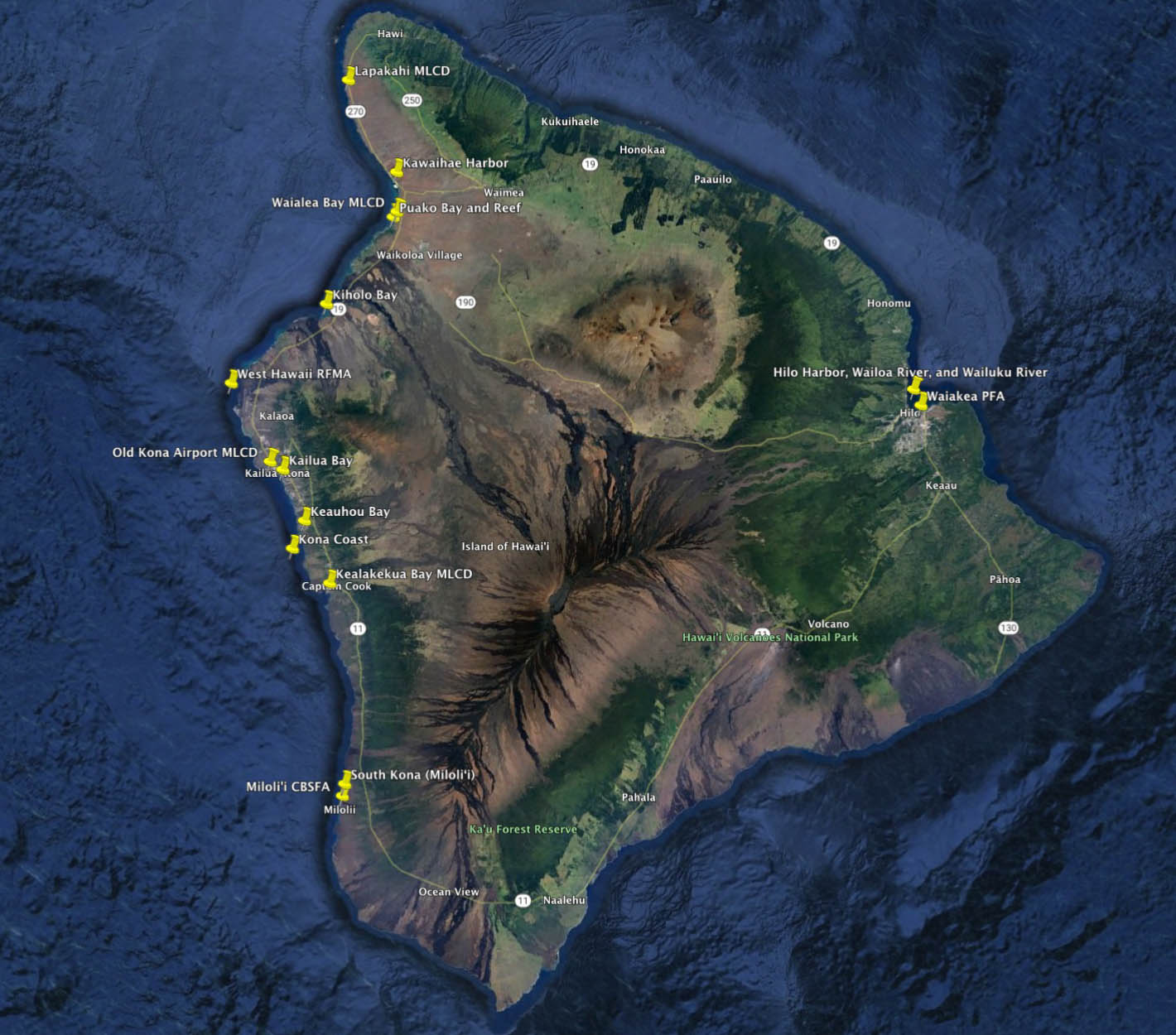This image is a detailed satellite view of the island of Hawaii, commonly known as the Big Island, surrounded by the dark, layered blues of the Pacific Ocean. The island itself is green, indicating lush vegetation, and brown in the center, reflecting the mountainous, volcanic regions, which include distinct craters or volcanoes. Its shape is irregular and roughly circular, with notable points and peninsulas. Roads, marked with white dots, meander along the coast and interior, and there are yellow pins highlighting key locations such as Hilo Harbor, Old Kona Airport, and Kealoha Bay. Labels on the map identify additional landmarks including Wailua River, Wailuku River, and South Kona, among others. This topographical map, resembling a Google Maps or MapQuest image, meticulously outlines both natural and man-made features, offering a comprehensive view of the island’s diverse landscape.